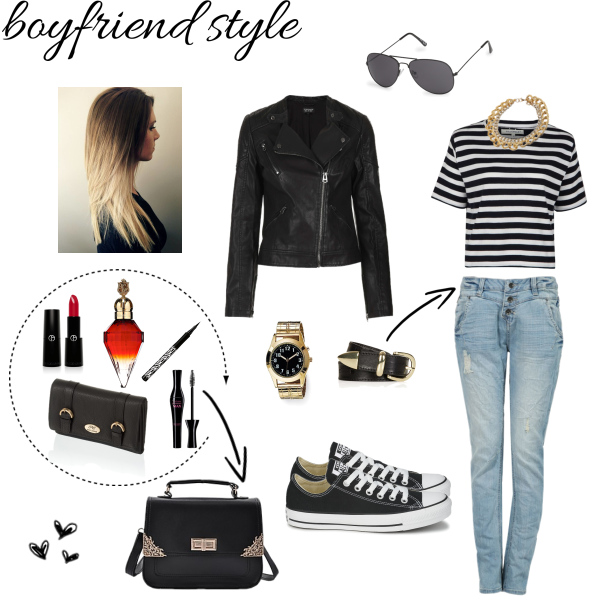In this image, labeled as "boyfriend style" in cursive black writing at the top left, various fashion items and accessories for women are artfully arranged against a white background. On the far right, a pair of aviator sunglasses points toward the bottom left. Beneath the sunglasses, a striped white and blue shirt is paired with faded skinny jeans and a necklace, possibly a choker. To the left of the shirt is a black leather jacket with a visible front zipper. Below the jacket, a gold watch with a black face can be seen, adjacent to a pair of black belts to the right. Additionally, there is a pair of classic Converse sneakers pointing to the right, located beside a black handbag adorned with metal fixtures.

A small, outlined circle with a dotted border contains various cosmetics, including lipstick, perfume in a red bottle with a gold cap, possibly mascara or eyeliner, and a pen. This circle is situated near a profile image of a woman with long, highlighted hair — blonde at the bottom and brunette at the top — wearing a black jacket or top. Her image is directly beneath the "boyfriend style" text. The collage is completed with three little black and white hearts drawn at the bottom left, adding a touch of whimsy. An arrow drawn from the belt points upwards and to the right, directing attention to the skinny jeans below the striped shirt.